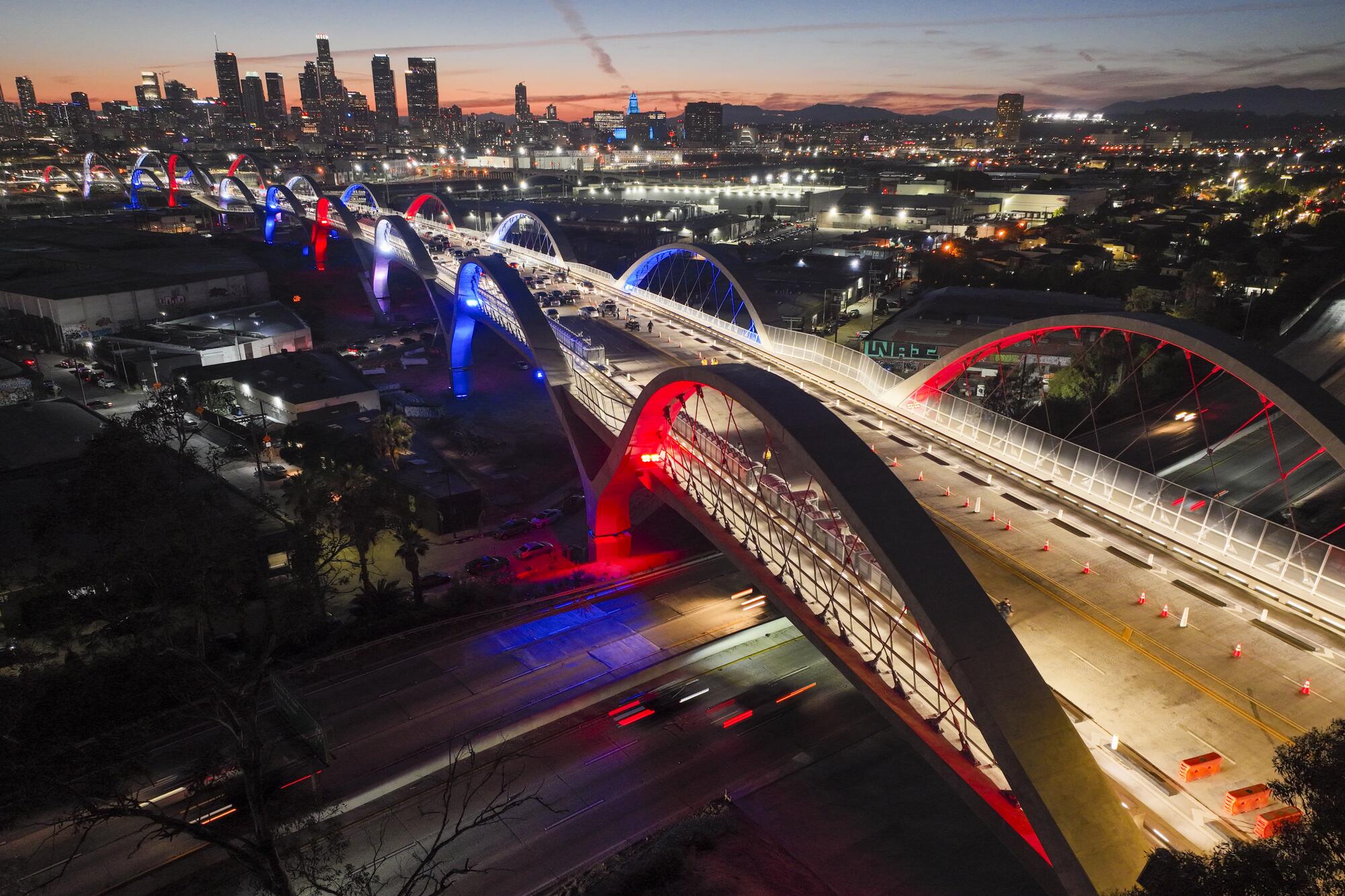The image captures a dynamic cityscape with a prominent bridge running diagonally from the bottom right to the top left. The bridge is wide and well-lit with patriotic blue, red, and possibly white lights illuminating its arches, creating a striking visual effect. In the foreground, the bridge appears empty, adorned with hazard cones, but further along, distant cars can be seen. Below the bridge, a bustling highway with visible traffic weaves through the city, accentuating the metropolitan setting. The backdrop features a diverse skyline—tall skyscrapers dominate the top left corner, tapering down to smaller buildings and residences toward the right. The sky, tinged with hues of gray, pink, and red, suggests a sunset, casting a warm glow over the scene. This image likely portrays a significant urban area, possibly resembling Los Angeles, capturing the transition from day to night in a city alive with lights and activity.